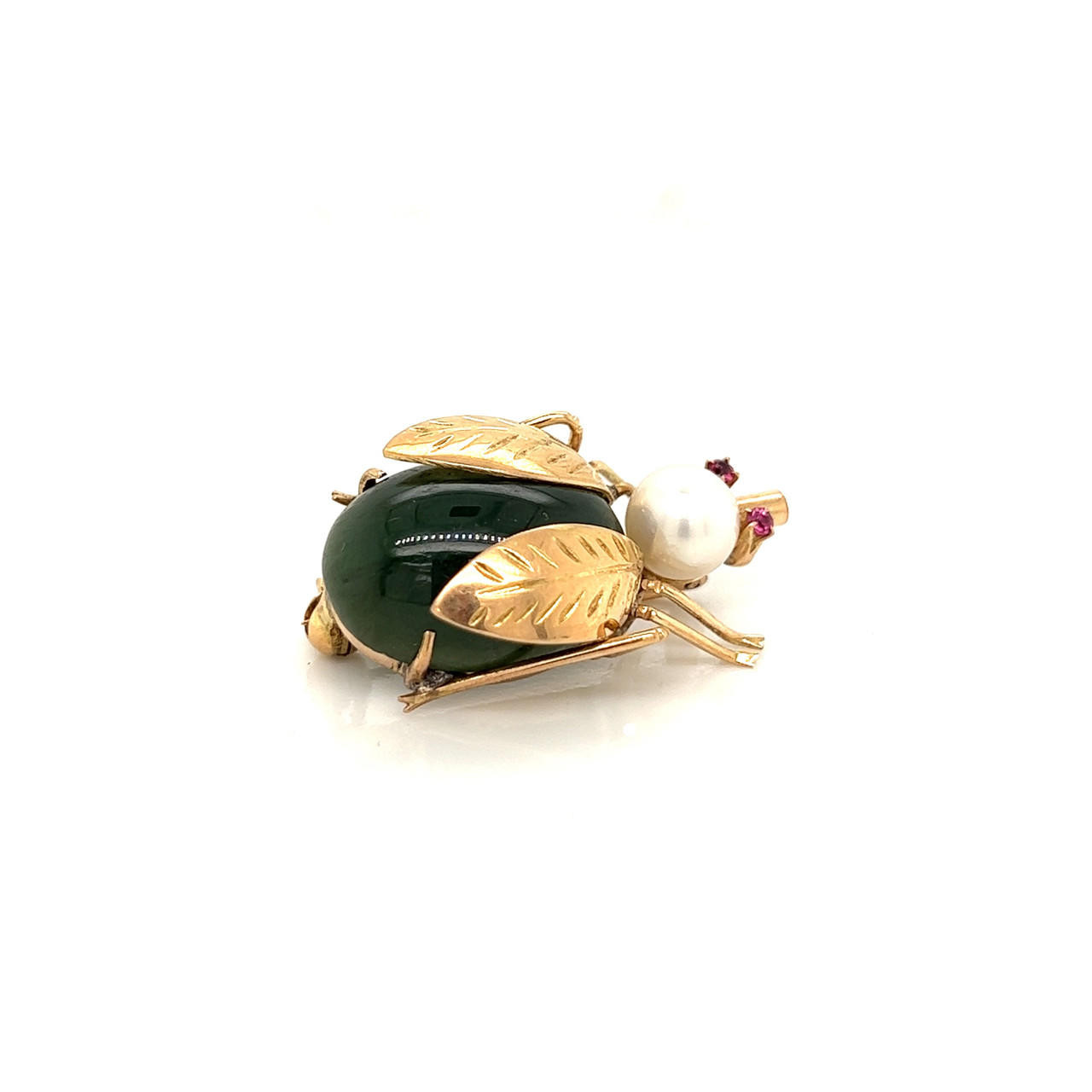This image features a detailed and exquisite insect-shaped brooch, likely intended as a decorative piece of jewelry. The brooch is designed to resemble a bee, with noteworthy elements that combine metal and gemstones. The body is composed of a well-polished, rounded green stone, resembling an emerald or jade, giving it a vivid, deep green hue. The bee's head is a lustrous white pearl, adding an elegant contrast. The insect’s wings are made of gold metal, intricately striated with lines to enhance their realistic appearance. Both its legs and tentacles are also cast in gold, complementing the golden wings.

Upon closer examination, there are tiny purple gems on either side of the bee's short snout, suggesting eyes, while a slight line of tiny white dots is visible along its back. The photograph captures the brooch against a white background, emphasizing the fine craftsmanship and ensuring that all details, such as the tube-like protrusion on its face and the compact nature of the piece (about the size of a coin), are clearly visible. This finely crafted brooch showcases a harmonious blend of materials and colors, making it a striking and well-kept piece of jewelry.